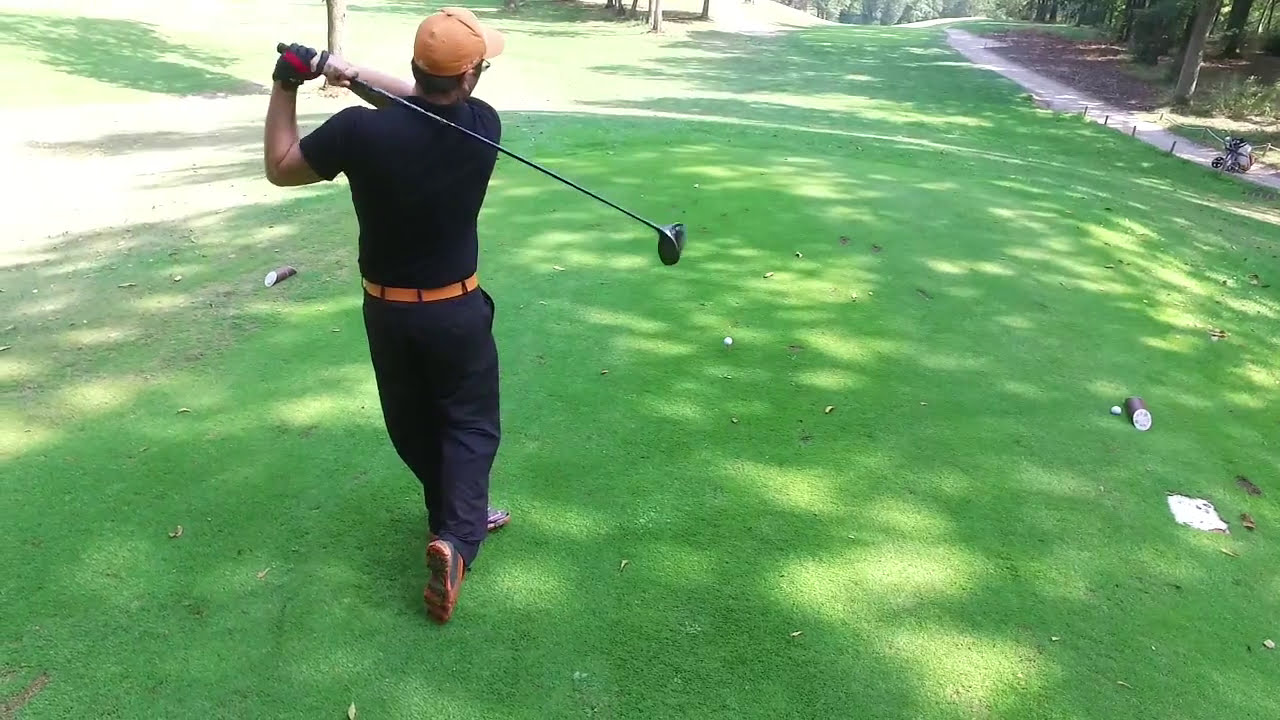This color photo, captured in landscape orientation by a drone, depicts a golfer mid-swing on a golf course. Positioned on the left side of the image, he has his club held high behind him, signifying a recent strike. The golfer's outfit is distinctive: he sports an orange cap, an orange belt, a dark blue shirt, black pants, and sneakers that are orange and gray. His hands are gloved in black gloves with magenta streaks. The ball he hit is visible a few feet ahead, while another lies near a container on the ground. The green includes some scattered golf accessories and debris. In the top right corner, a paved path with a baby carriage, or two-wheel hand cart, is noticeable. Large trees loom beyond the path, bathed in what appears to be the gentle light of early evening, enhancing the realistic, representational style of the photograph.